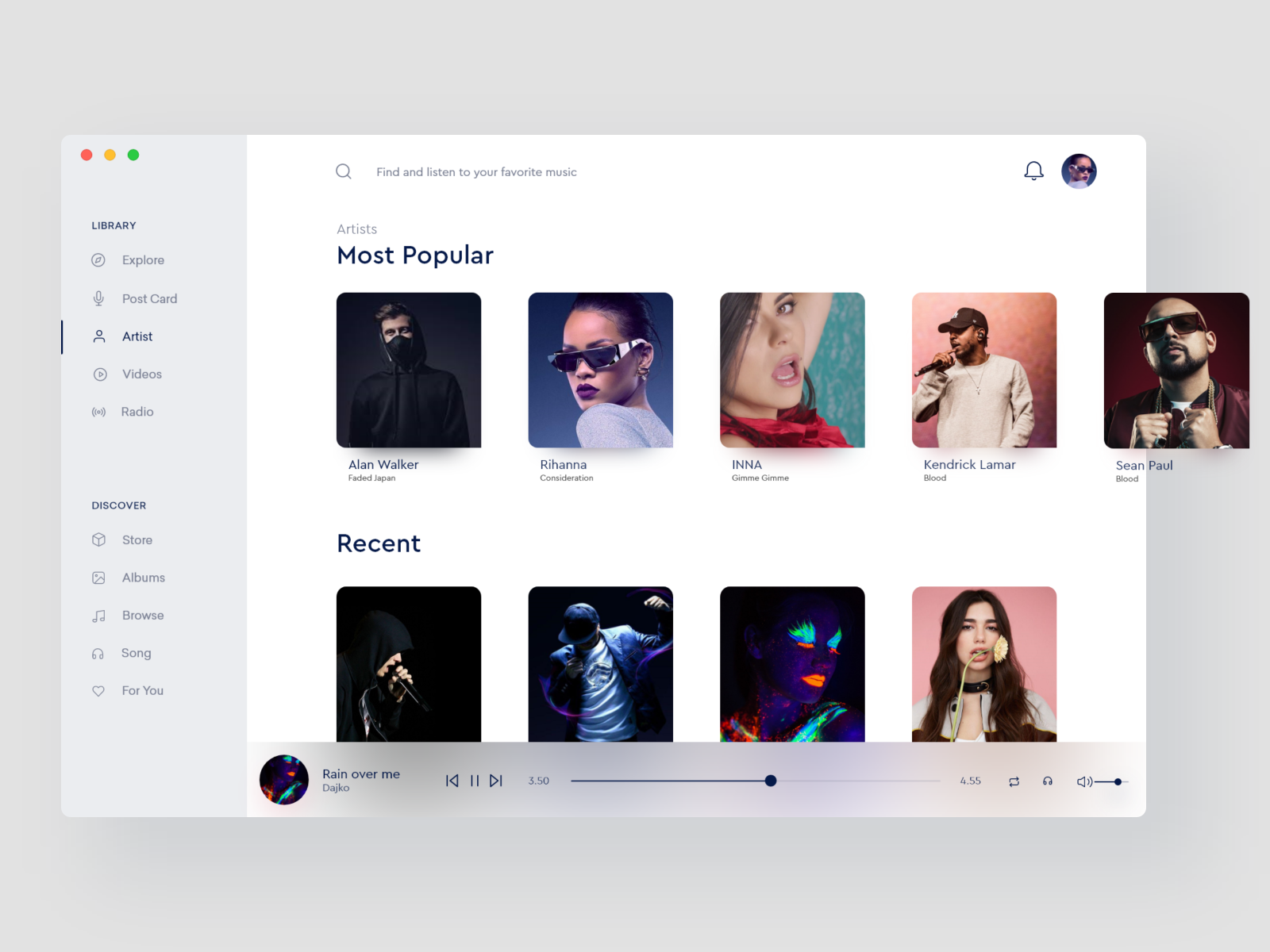This image depicts the user interface of an Apple Music or iTunes library on a Mac computer. The screen showcases the homepage dedicated to artists, featuring a sidebar on the left with a gray background that lists various sections including 'Library,' 'Explore,' 'Postcard,' 'Artist,' 'Videos,' and 'Radio' in a vertical arrangement.

To the right of the sidebar, additional categories such as 'Discover,' 'Store,' 'Albums,' 'Browse,' 'Songs,' and 'For You' are displayed. The main focus of the image is a track playing screen, currently showing the song "Rain Over Me" by Dashco at the 3-minute and 50-second mark of a total duration of 4 minutes and 55 seconds. Below this is the playback control panel, including buttons for replay, pause, and fast forward. There's also a shuffle button located on the right-hand side of the song duration indicator. Additionally, a headphone icon suggests connectivity options, and a volume scrollbar is present for adjusting the sound level.

In the central part of the interface, a section titled 'Artists Most Popular' is visible, featuring prominent artists such as Alan Walker, Rihanna, Inna, Kendrick Lamar, and Sean Paul. Accompanying this is a 'Recent' section that displays other artists like Eminem among others. Each artist entry is represented with distinct cover art. For instance, Rihanna is depicted wearing sunglasses and a light purple long-sleeve shirt with matching purple lip gloss, while Alan Walker is shown in a blacked-out hoodie and a black KN95 mask, revealing only his eyes, forehead, and hair.

At the top right, there is a profile icon that mirrors Rihanna's cover art but positioned slightly differently—her gaze is directed to the right instead of the left, although she is dressed in the same outfit.